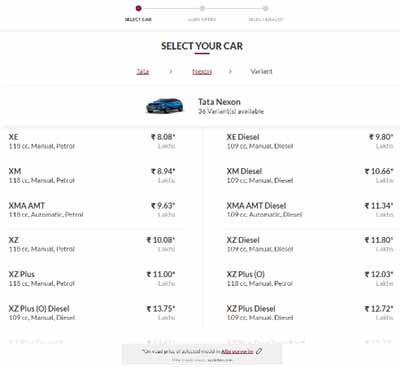On a car dealership website, the user is prompted to select their preferred car model. The screen displays the Tata Nexon with its image prominently featured. Below the image, there's a list detailing various customization options, such as choosing between a manual or automatic transmission, and selecting fuel types like diesel. These selections are accompanied by values in an unfamiliar currency, indicating additional costs for each feature. The page is designed to guide the user through the car customization process, represented by a status bar at the top, indicating that they are currently on step one of three in the configuration process. Further steps require the user to sign up or log in to proceed.